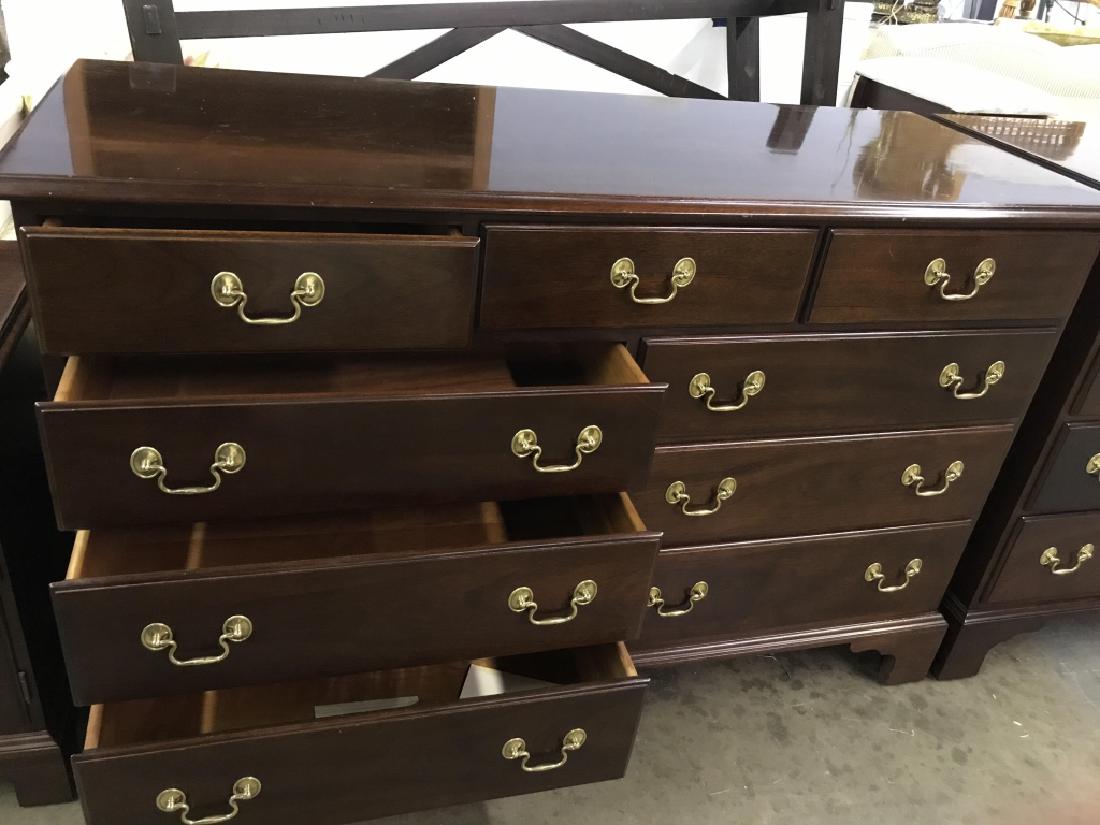The image displays a dark-stained wooden chest of drawers, featuring a high-gloss sheen on its top surface, suggesting a polished finish. This chest is comprised of four rows with a total of nine drawers: the top row houses three smaller drawers, each with a single brass handle, while the three subsequent rows contain larger drawers, with two brass handles each. The legs elevate the chest above a concrete pad, and the brightly illuminated surroundings imply daylight conditions, possibly outdoors or in a well-lit warehouse or storage facility. Left-side drawers are slightly open, revealing a lighter wood interior, contrasting the darker exterior. The scene includes additional furniture pieces in the background, such as a possible headboard and the edge of another dresser, lending an impression of a furniture display or storage setting.